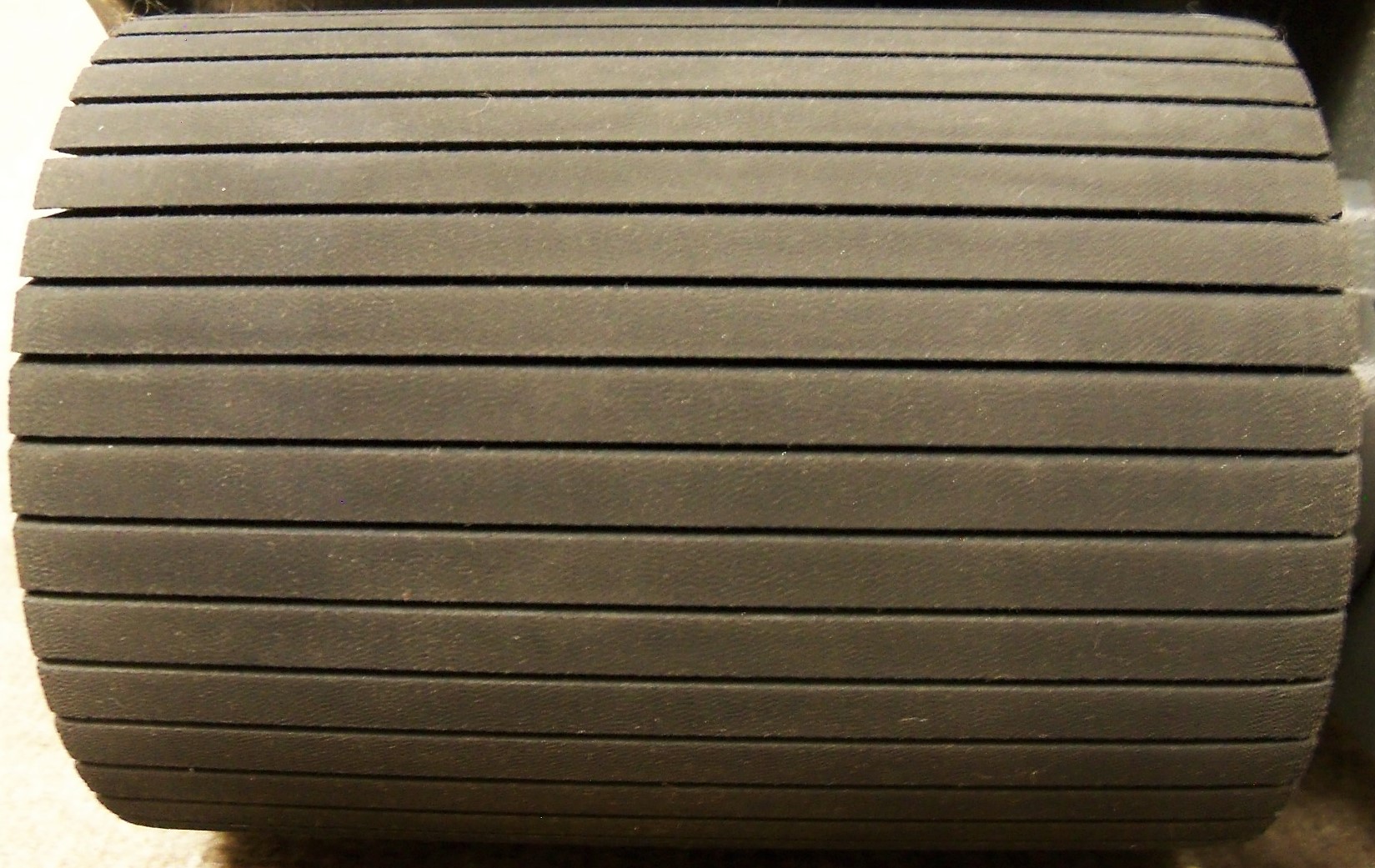This detailed close-up photograph depicts a dark, possibly black or dark gray cylinder occupying nearly the entire frame, stretching from left to right and top to bottom. The cylinder features dark gray or blackish slats arranged in a uniform pattern with gaps between them. These slats appear aged, with visible dust or dirt, suggesting significant usage, possibly being rolled across the ground repeatedly. The edges of the slats are slightly more frayed and worn than the central parts. The material, although dark in color, is hinted to be brown by one observer. The image provides no context or background details, and no text is visible. It could be a close-up of a fabric or material wrapped around a metal rod, potentially part of a production line or conveyor belt setup, but the precise nature of the object remains unclear due to the tight framing of the photograph.